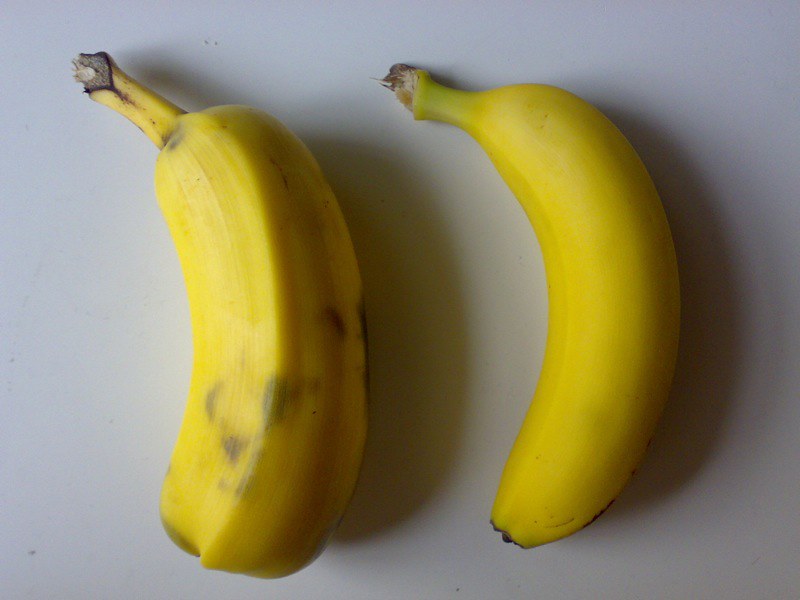The image showcases two bananas side by side, clearly from different varieties. The banana on the right is the classic variety typically found in the UK, with a bright yellow peel, a slightly green stalk, a small brown mark on the side, and a uniform shape free from bruises – it appears perfectly ripe and ready to eat. 

In contrast, the banana on the left seems to be a different variety altogether. It features a distinctive circular cap where it joins the stalk and is significantly thicker than its counterpart. This banana exhibits various unusual markings, including several dark black dents, a brown dent, and a few green and black dents on the front. A prominent rib runs down the center of its peel, which is not seen on the other banana. Despite being of similar length, the banana on the left looks as if it might be only half a banana due to its substantial girth, highlighting the stark difference between the two.